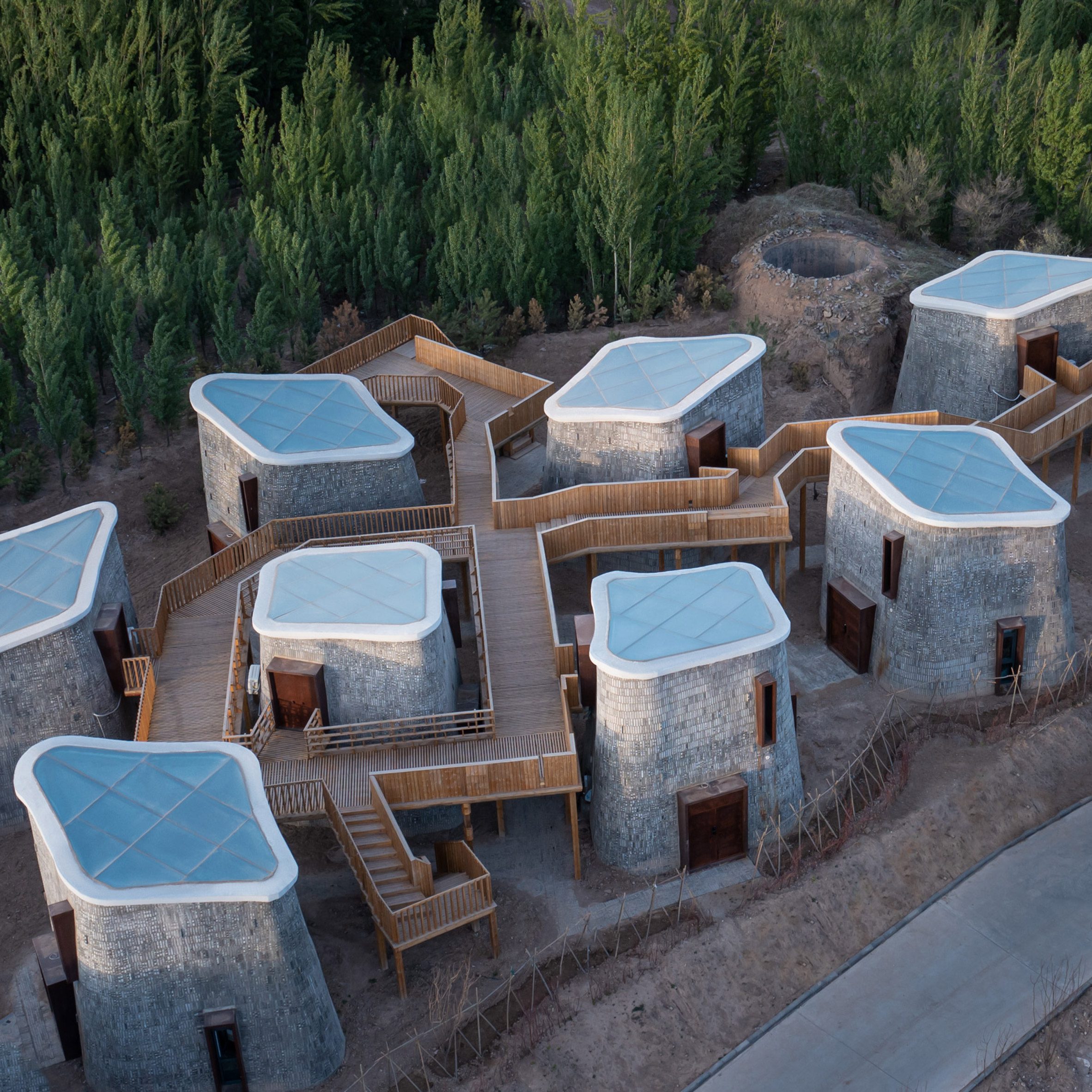This image depicts a primitive yet futuristic-looking village from an aerial perspective. The village consists of eight closely arranged two-story townhouses made of light bricks or stone. Each building features a quilted gray, diamond-shaped, or rhombus-like flat roof that appears to be solar-paneled and is framed with white guttering. These structures are interconnected by a wooden walkway or boardwalk on the second level, providing access to each home. The buildings have uniform windows and doorways: a long, narrow top window and two large double doors at the lower level. 

In the foreground, a staircase descends from the elevated walkway to the ground, which is a mixture of tan and brown shades, resembling dirt or hay with no visible grass. A paved roadway runs diagonally from the middle lower edge to the lower right corner of the image. The background is filled with dense, large green trees and smaller bushes, creating a natural perimeter around the village. Additionally, a round, hollow structure is noticeable in the background, contributing to the scenic and detailed composition of this primitive yet modernized village.